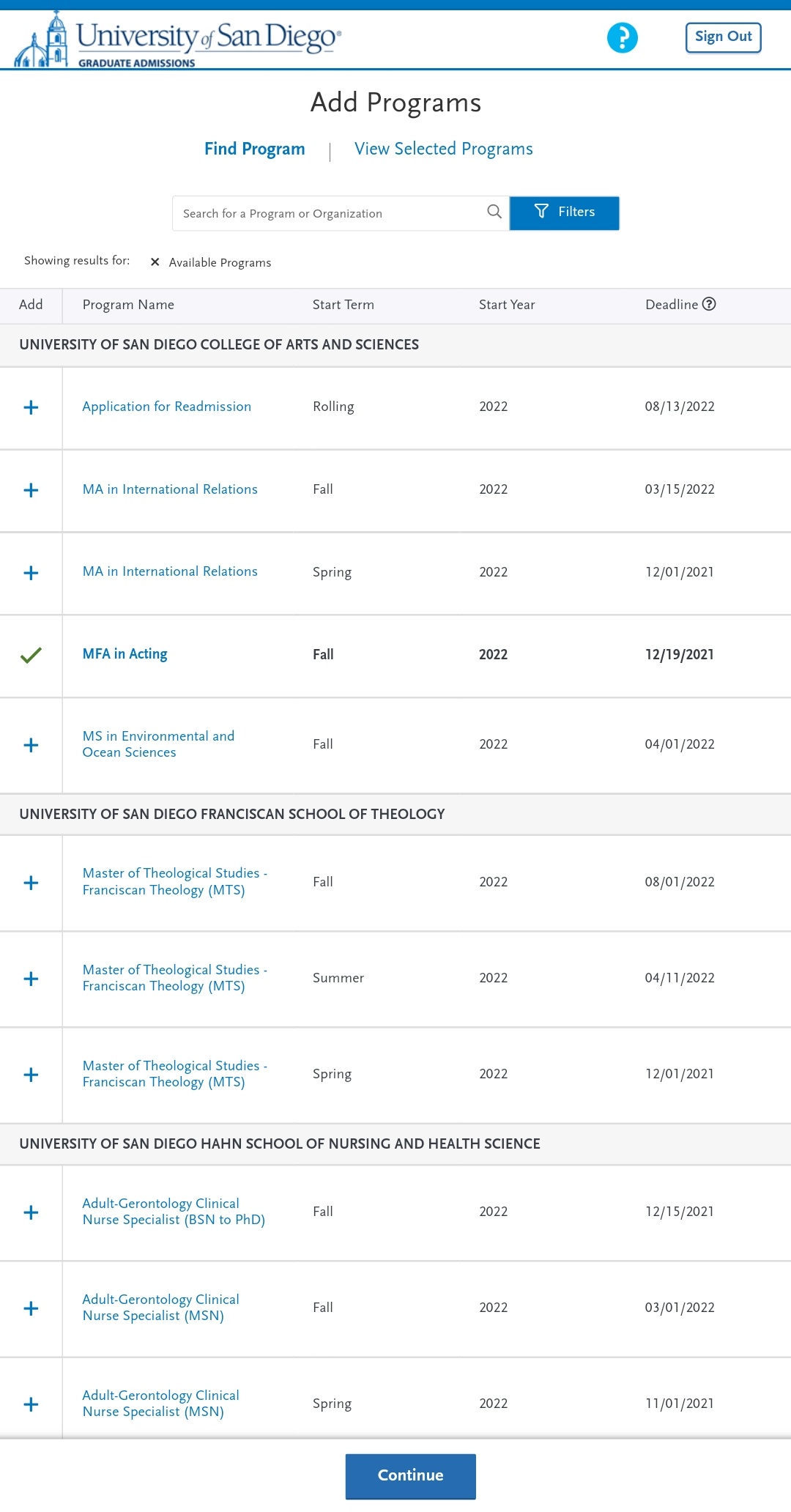A detailed caption for the image described could be:

---

This screenshot, captured from a mobile device, showcases the "University of San Diego" website, specifically the "Graduate Admissions" section. The top banner displays the university's name along with a blue question mark icon on the left side and a blue "Sign Up" button on the right. Beneath the header, there are several options: "Add Programs," "Find Program," and "View Selected Programs." Below these options, a search bar accompanied by a blue "Filters" button allows users to refine their search queries.

The search results display a list of available programs at the university. It indicates "Showing results for available programs" and presents data in a tabular format with columns titled "Add," "Program Name," "Start Term," "Start Year," and "Deadline." Three schools within the university are listed with respective program information:

1. University of San Diego College of Arts and Sciences
2. University of San Diego Franciscan School of Theology
3. University of San Diego Hahn School of Nursing and Health Science

Each school entry includes details about the programs they offer. At the bottom of the screen, a prominent blue "Continue" button allows users to proceed with their selections. The overall color scheme of the website is primarily blue and white.

---

This caption comprehensively describes the layout, content, and functionality of the webpage, providing a clear understanding of the image.